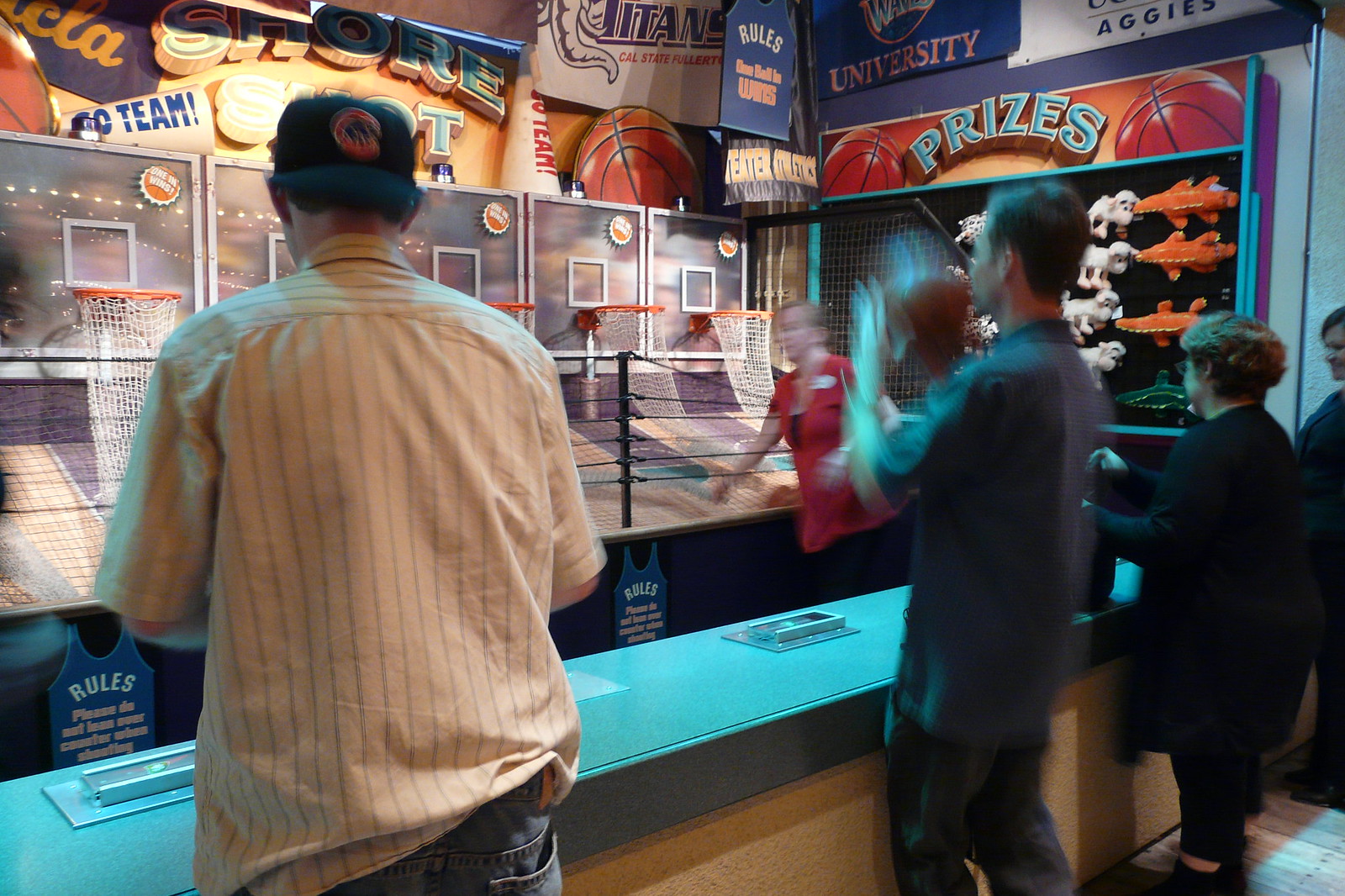The image captures a lively scene at an indoor arcade, centered around an arcade basketball game. Prominently featured is a blue and beige counter where participants line up to take their shots. To the left, a man stands with his back to the viewer, identifiable by his backwards baseball cap, white and blue striped short-sleeved dress shirt, and jeans. Beside him, another man with short, dark hair is caught mid-action, throwing a basketball; he's wearing a blue shirt and jeans. Next to him, a child with short brown hair, dressed in a long shirt and pants, also engages in the game.

On the right side of the image, partially obscured by players, an attendant in a red vest layered over a black sweater stands near a prize display case. She has a white name tag pinned to her vest. Above her, the word "PRIZES" is clearly visible, hinting at the arcade's reward system. The display case showcases an array of stuffed animals, including sheep, spotted creatures, orange alligators or dinosaurs, sharks, and dogs.

The back wall of the arcade, decorated with small basketball hoops, features motivational words like "SHORE," "SHOT," and "GO TEAM," along with a large basketball graphic. There is also a partial view of a sign marked "RULES," though the details are unreadable. The scene is a snapshot of the fun and excitement typical of an arcade environment.